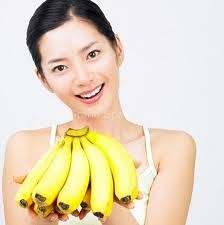The image captures a young Asian woman with dark hair pulled back, her head tilted to the right (left side of the image). She is wearing a white spaghetti-strap tank top that reveals her bare shoulders and slim frame, highlighted by her pronounced clavicle. Her parted hair falls to the left side of her head (right side for the viewer), and her complexion is a light ivory. The woman, adorned with dark eyebrows, dark brown eyes, and pink lipstick, is smiling broadly, showcasing her white teeth. Cradled in both her palms in front of her chest is a bunch of ripe, yellow bananas, with some having little black tips visible. The photograph, featuring a crisp white background, ends around her forearms. A faint, illegible white watermark is visible just below her chin. The overall dimensions of the image are small, almost square, and the bright lighting creates a soft white shadow on the bananas.